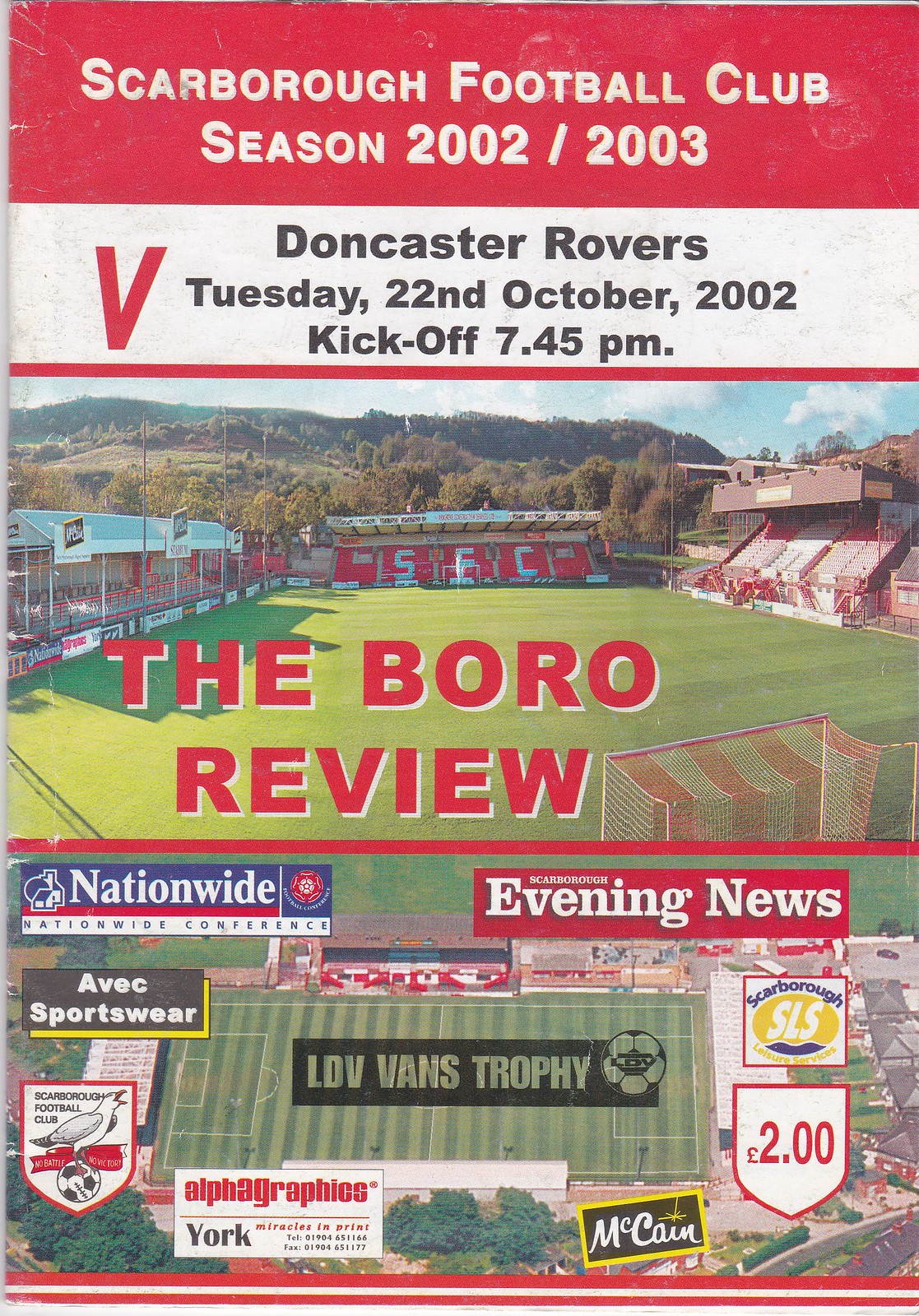This image is of a vintage, event program or poster for a football (soccer) match. At the very top, a red rectangular banner bears the title "Scarborough Football Club Season 2002/2003" in white letters. Directly below is another section listing the match details in black font: "Doncaster Rovers, Tuesday 22nd October 2002, kick off 7.45 p.m." Central to the image is a colored photograph depicting a soccer field flanked by bleachers on the left, right, and back sides. Prominently displayed in red, capital letters is the section title "THE BOROUGH REVIEW." At the bottom of the poster, several advertisements from sponsors such as Nationwide, Evening News, Avec Sportswear, LDV Vans Trophy, AlphaGraphics, McCain, and other companies decorate the image. The overall design and details indicate it is from approximately 20 years ago, likely emphasizing the nostalgic aspect of the event.